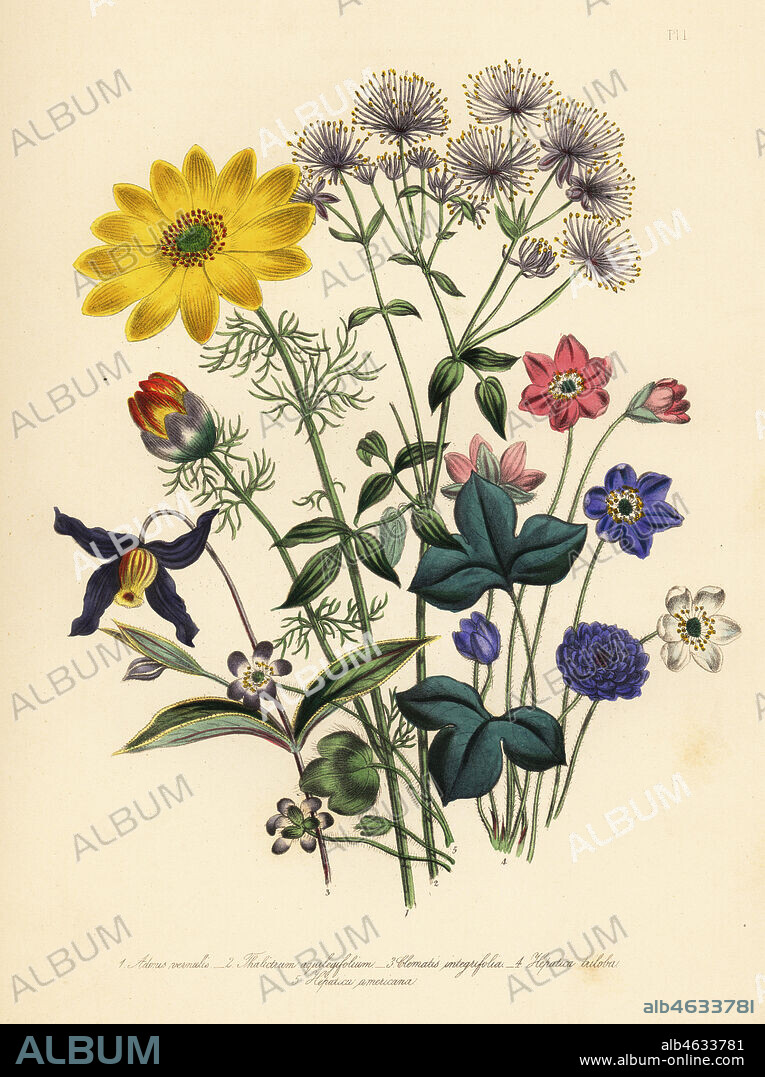This botanical image is a detailed stock photo showcasing a variety of colorful flowers set against a cream or beige background that resembles old historic paper. The background is repeatedly watermarked with the word "album" in a vertical pattern. At the very bottom of the image, a black stripe features the text “album” alongside a serial number “alb4633781” and a website “www.album-online.com.” The floral arrangement includes approximately ten different types of flowers, with notable examples such as a yellow flower with a green center, a blue flower with yellow accents that comes in pinkish-red and white variations, and a tulip-like flower in red, yellow, and purple hues. The flowers are rendered to mimic hand-colored watercolor illustrations.